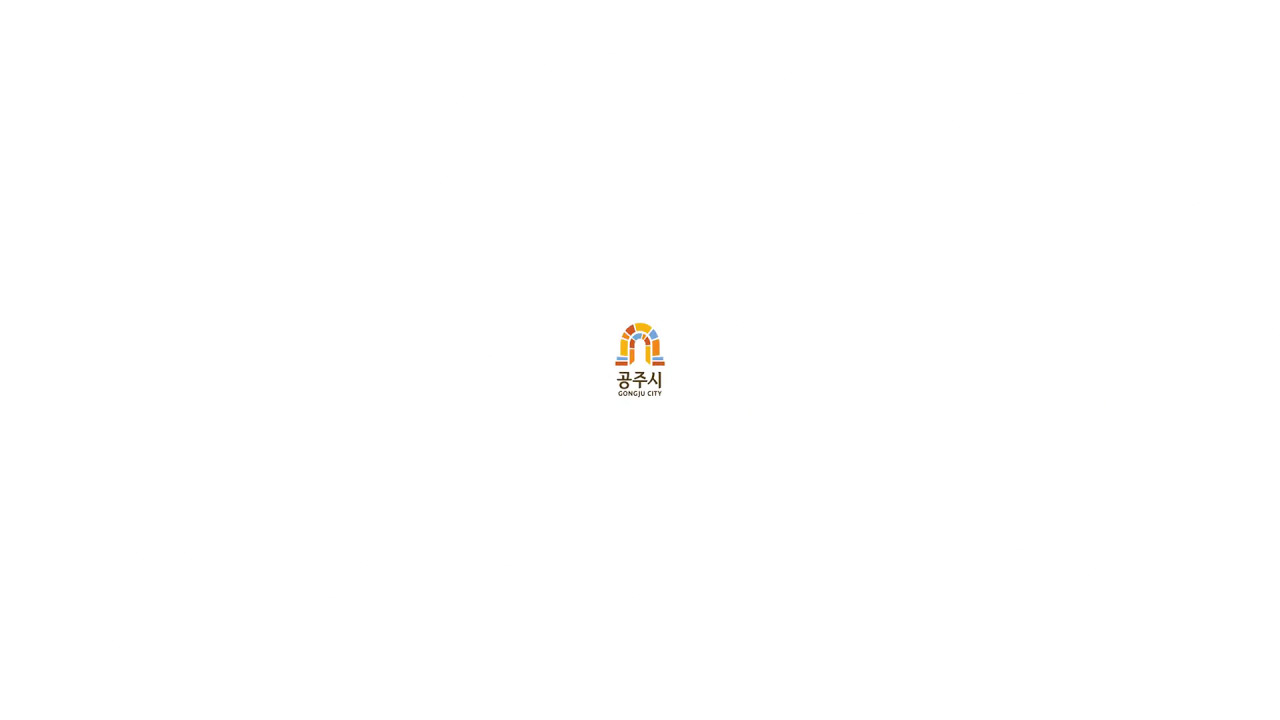The image shows a simple logo centered against a solid white background, devoid of any borders or additional objects. The logo itself resembles an upside-down U-shaped archway, imbued with a gradient of colors starting from a red base, transitioning through blue, orange, darker orange, yellow, and ending in blue. Within this archway, a smaller archway is nested, possibly suggesting depth or distance. Below the archway symbol, there are two lines of text. The top line features Asian characters, likely Korean, and the bottom line reads "Gongju City" in brown letters. The text and logo are positioned centrally, emphasizing a minimalistic and clean aesthetic that could be fitting for a company logo, possibly featured on materials like business cards.